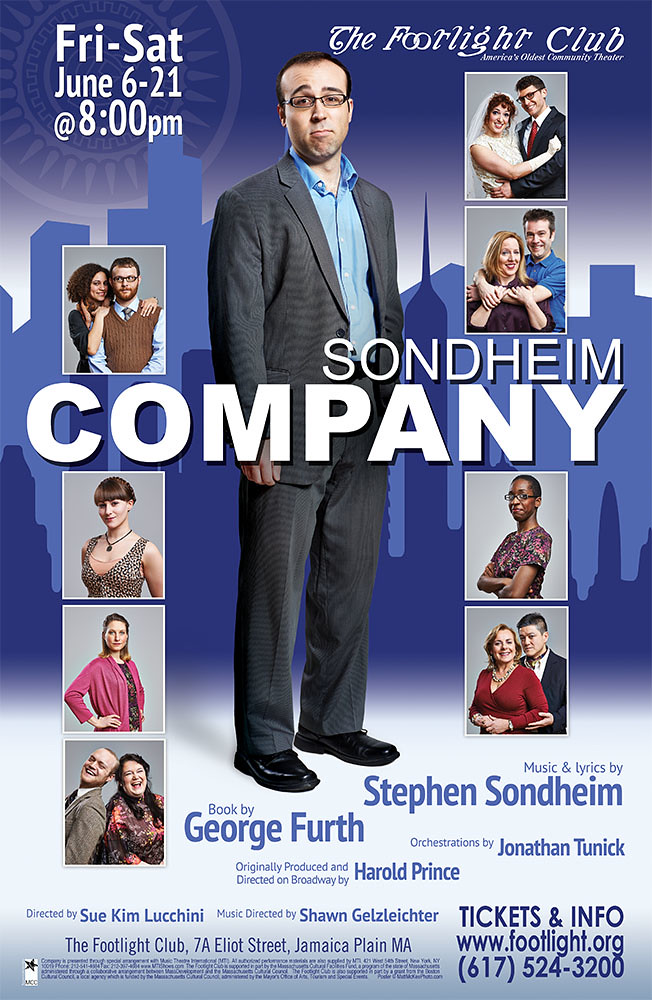The poster for the play or movie prominently showcases a man in a gray suit and glasses standing at the center, looking perplexed. This is framed by several small, white-bordered portrait photos on either side. In the first row of photos on the left, there is a man with his bride, a man and woman with the man embracing the woman from behind, and a lone woman in a spotted dress with brown hair and a black necklace. Below these images are a young African American woman with arms crossed, another woman in a pink sweater with hands on her hips, and a couple with the man in a black suit and the woman in a red dress. The right side mirrors this with photos of another couple smiling and laughing, a lone woman in a floral or abstract pattern shirt, and another woman by herself. 

At the top right corner in large text, it reads "The Footlight Club," noted as America's oldest community theater. The central text exclaims "Sondheim Company" in bold white letters. Event details are provided at the top left, stating "Friday through Saturday, June 6th to 21st, 8 p.m." 

The background is a stylized cityscape in varying shades of blue and dark blue, with the skyline appearing two-dimensional. The gradient sky transitions from dark blue at the top to a lighter hue closer to the skyline and eventually white near the ground. At the poster's bottom, additional text provides critical details: 

"Music and Lyrics by Stephen Sondheim
Book by George Firth
Orchestrations by Jonathan Tunick
Originally produced and directed on Broadway by Harold Prince
Directed by Sue Kim Luchini
Music directed by Shawn Gelsleichter"

Ticket information, including the website www.footlight.org and phone number 617-524-3200, is positioned in the corner, along with a star icon denoting more details too small to read. The cityscape background continues behind the text, transitioning to a lighter blue at the bottom, creating a visually cohesive design.